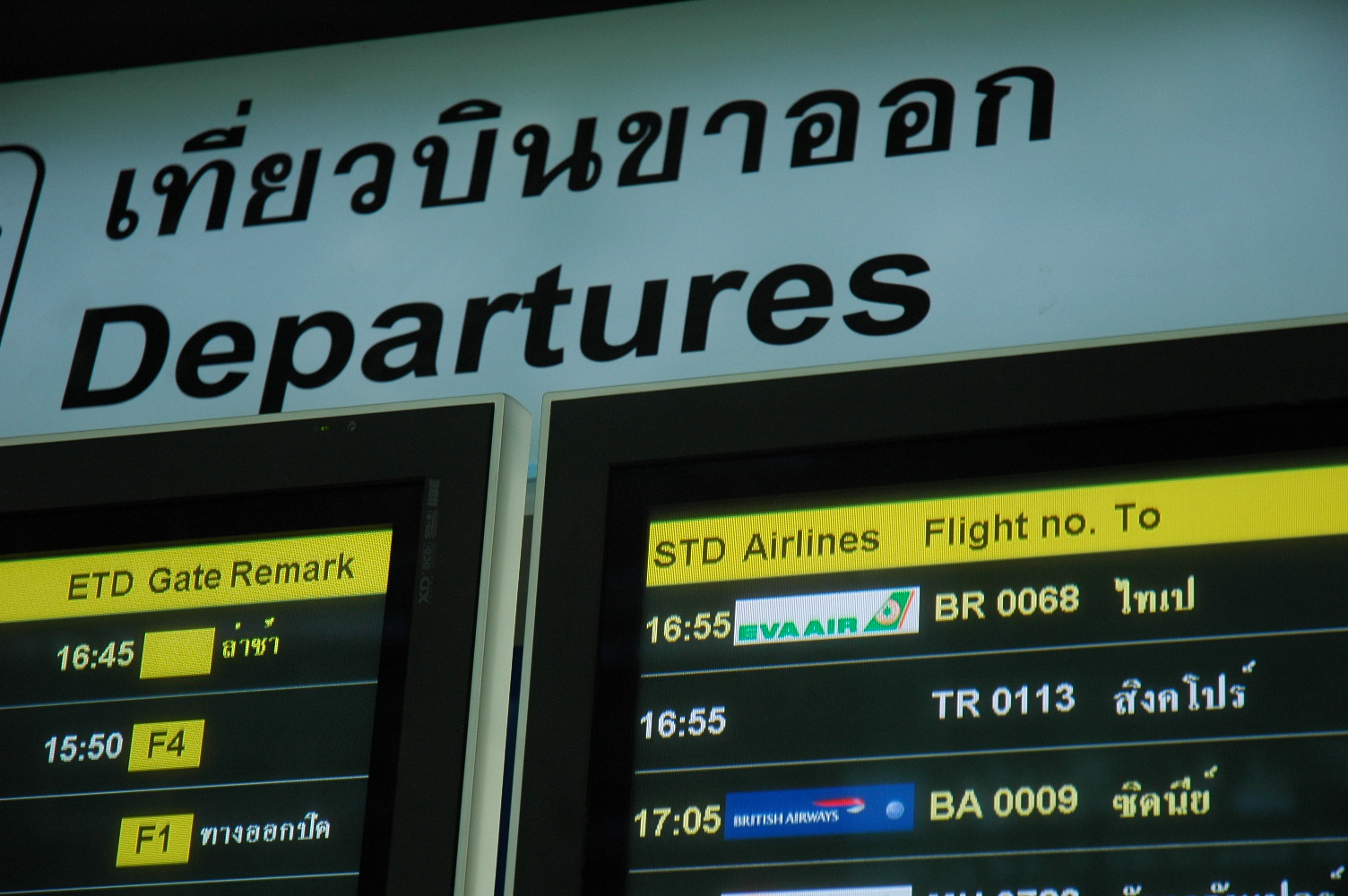The image depicts a pair of airport departure boards, prominently situated to display flight information in both a foreign language—possibly Arabic or an Indian script—and English. The top of the boards features a white banner with the word "Departures" in bold black letters, mirrored by the foreign language text above it.

The screen on the right includes a yellow banner header with columns labeled STD (Scheduled Time of Departure), Airlines, Flight Number, and To. Below this, the Airlines column features the logos of EVA Air and British Airways, accompanied by their respective flight numbers: BR 0068, TR 0113, and BA 0009. The times are indicated in a 24-hour format: 1655, 1655, and 1705, respectively.

On the left screen, a similar layout is found, with columns for ETD (Estimated Time of Departure), Gate, and Remarks. The ETD column lists the departure times 1645 and 1550, with corresponding gate numbers F4 and F1, while the Remarks column is filled with text in the same foreign language.

Both screens utilize a combination of yellow and white text on a black background to clearly present vital travel information, ensuring clarity and efficiency for travelers.